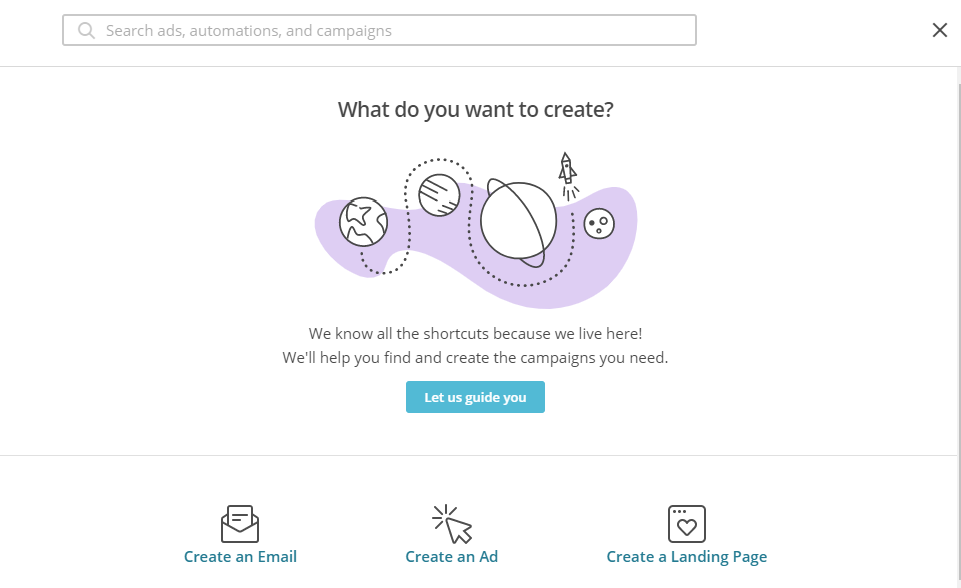The image depicts a vibrant website interface designed for managing digital marketing tasks. At the very top of the screen, there is a search bar labeled "Search ads, automations, and campaigns," providing users with a straightforward way to navigate the platform's features. In the upper right corner, there's an "X" icon to close the current screen.

Dominating the center of the image is a motivational prompt that reads, "What do you want to create?" Accompanying this text is a dynamic graphic of a rocket ship soaring through space, having departed from Earth and navigating past celestial bodies including Saturn and the Moon. The imagery emphasizes the theme, "We know all the shortcuts because we live here. We'll help you find and create the campaigns you need. Let us guide you." Notably, the phrase "Let us guide you" is highlighted within a blue rectangle to draw attention.

Towards the lower section of the image, there are three distinct action prompts each accompanied by an icon. On the lower left, there is an option titled "Create an email," depicted with an envelope icon featuring a letter partially out of it. The middle section presents the option "Create an ad," symbolized by an arrow icon with a starburst effect at its tip. Finally, in the lower right, there's an option to "Create a landing page," illustrated with a square icon featuring three dots in its upper left corner and a heart shape within.